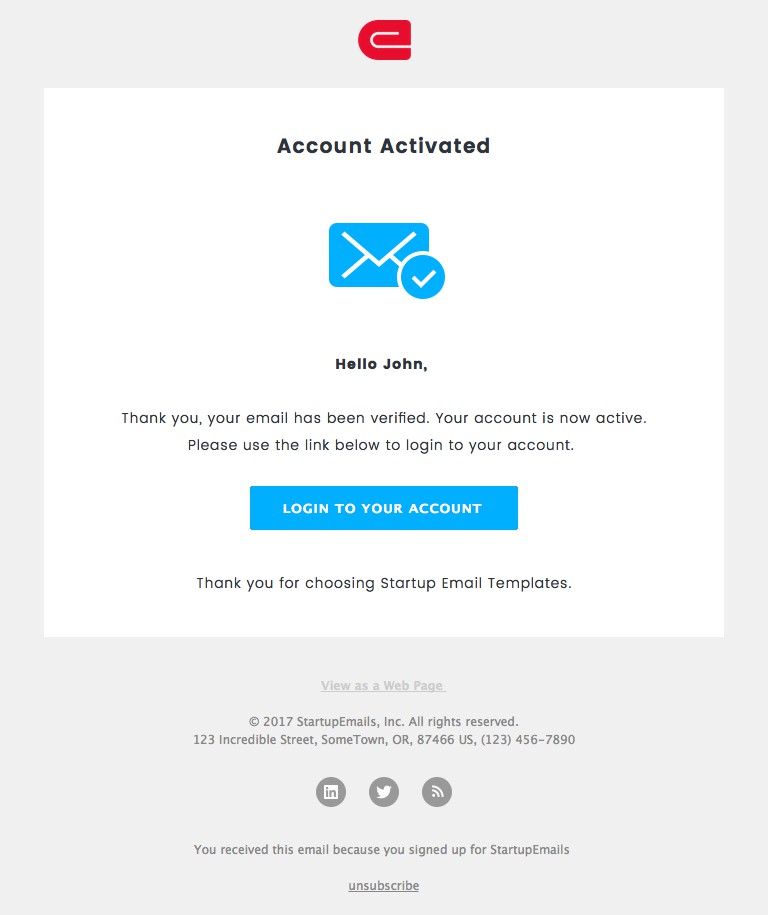This screenshot captures an email sent from an unidentified brand, distinguishable by a red, lowercase 'e' logo. The email, addressed to a person named John, confirms that his email has been verified and his account is now active. To log into his account, John is prompted to use a prominently displayed blue button provided within the email. 

The message expresses gratitude for choosing "Startup Email Templates" and includes an option to view the email as a webpage for a more enhanced visual experience. At the bottom of the email, there is a standard copyright notice from 2017 attributed to "Startup Emails Inc.," located at 123 Incredible Street, Sumtown, Oregon, 87466, USA, along with a generic contact number.

Additionally, the email contains social media icons directing users to the company's LinkedIn and Twitter profiles, as well as an unidentified icon resembling a diagonally positioned Wi-Fi symbol. Finally, the email informs recipients that they received this communication because they signed up for "Startup Emails," and provides an option to unsubscribe.